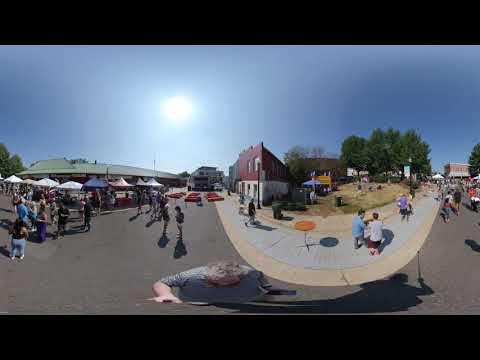The image portrays a bustling outdoor scene on a sunny day, likely a community event or market in a small southern town. Under a clear blue sky, around 20 people meander along a road flanked by a variety of colorful umbrellas—white, blue, and more—providing shade to the stalls beneath. On the left-hand side, a small building with a green awning stands near the line of umbrella-covered stalls. To the right, a two-story building catches the eye; its lower half is painted white, while the upper portion is red. In front of this building, a wide sidewalk extends toward the camera and loops further right, framing some large bushy trees and revealing a red-brick corner store in the distance. Amongst the crowd are people in casual attire, including a woman in jeans and another in purple pants, suggesting a relaxed atmosphere. The historic architecture of the buildings, reminiscent of the 1800s, and the organized setup with tents hint at a well-planned community event, likely sanctioned by the city council. The scene is lively, with families and individuals enjoying the pleasant day.